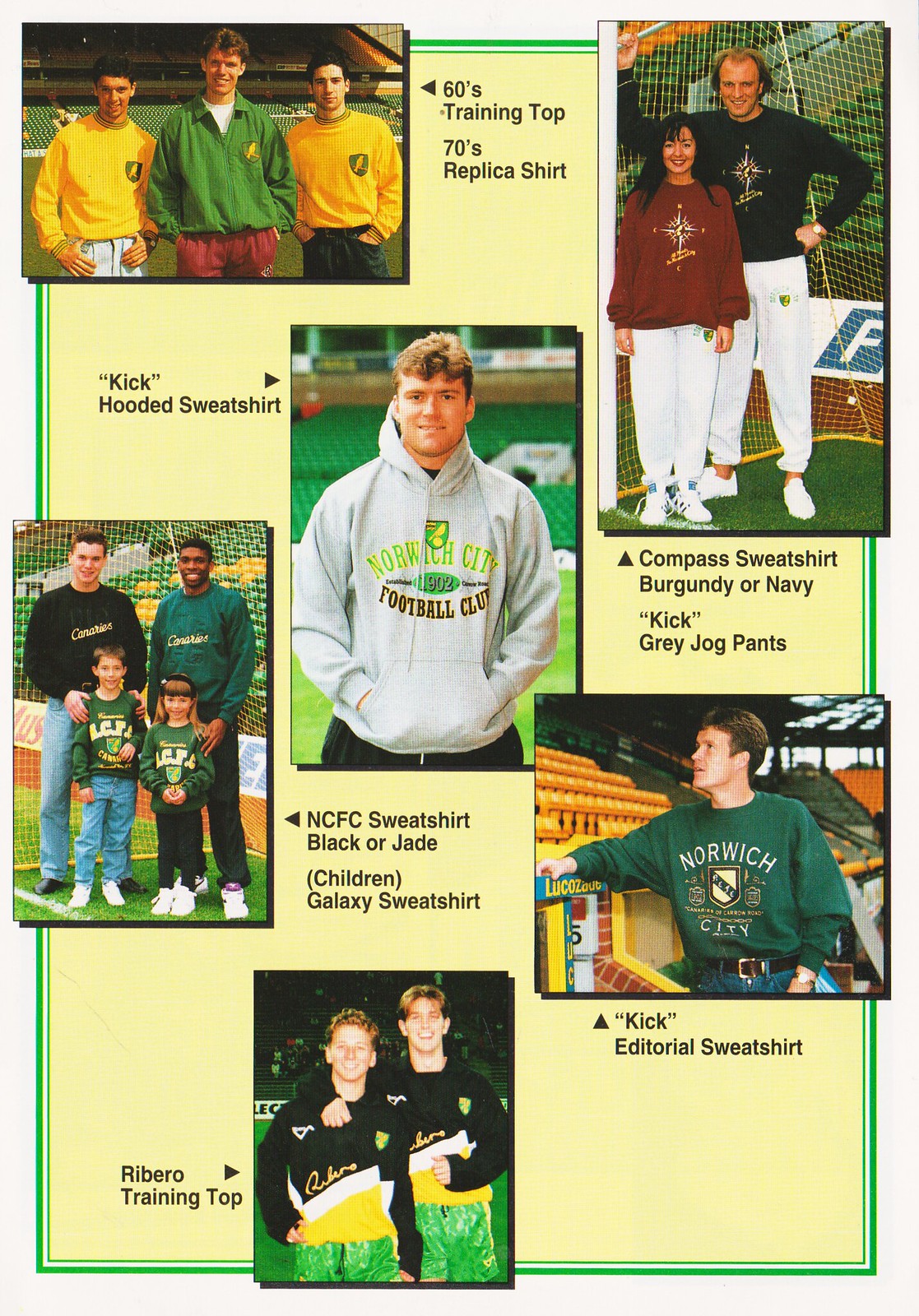The image is a meticulously arranged graphic collage with a neon green border, containing a collection of photographs and labels that showcase various people modeling sportswear through the years. Central to the image is a male figure donning a white or gray hoodie labeled "Kick Hooded Sweatshirt." Above him, on the upper left, three men stand side by side on a field, clothed in retro sportswear: two in yellow long sleeves and one in a green long sleeve, collectively captioned "60s Training Top, 70s Replica Shirt."

To the right of this trio, a man and a woman pose in long-sleeved sweatshirts—hers red and his black—paired with white jog pants; the label beneath reads "Compass Sweatshirt, Burgundy or Navy, Kick Gray Jog Pants." Below these images, a group photo features two adults and two children wearing logoed sweatshirts: the adults in black and green, and the children in matching jade tops. The caption here reads "NCFC Sweatshirt, Black or Jade, Children Galaxy Sweatshirt."

Further to the right, a solo image spotlights a man in a green sweatshirt, marked "Kick Editorial Sweatshirt." Wrapping up the montage, at the bottom left, two men sport black and yellow tops, identified as "Ribeiro Training Top." This collection of images appears to be an elaborate catalog for a sports team or brand, presenting a range of apparel from various decades.